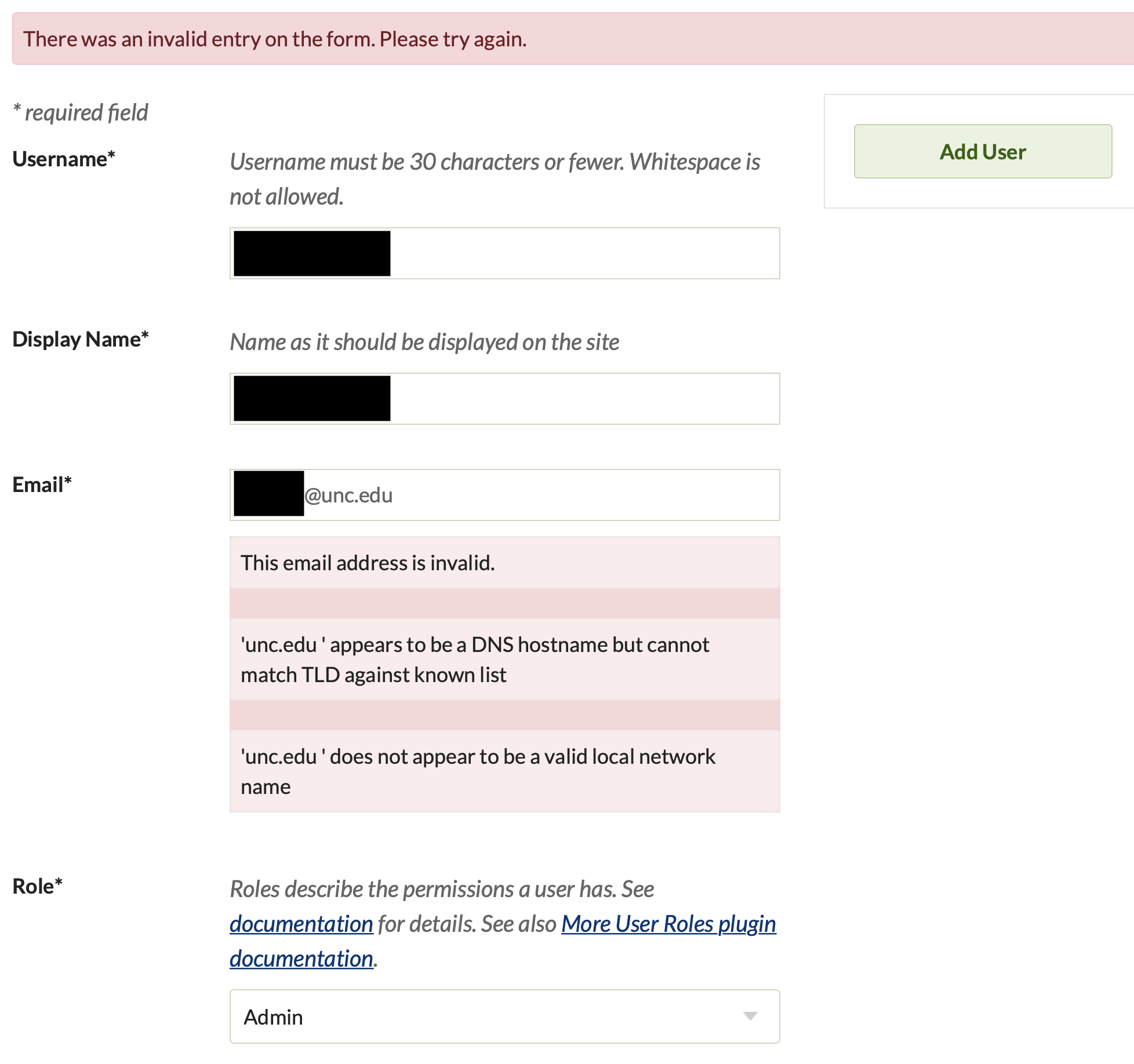**Caption:**

This screenshot displays a form from a web page with several fields and prompts for user inputs. 

1. At the very top, there is a prominent pink rectangular notification box containing a warning message in red letters that reads: "There was an invalid entry on the form. Please try again."
2. Below this warning, a required field is indicated with an asterisk.
3. On the left-hand side, the form requests a "Username" followed by an asterisk to signify its necessity. The note beside it specifies, "Username must be 30 characters or fewer. White space is not allowed."
4. Next to this note is a long rectangular input box, partially filled with black, indicating a potential entry, while the rest of the input area is blank.
5. To the right of this username input field is a green "Add User" button.
6. Directly beneath the username section, the form prompts for a "Display Name," meant for the name's appearance on the site. This is followed by another long input box that's half white and part black.
7. The form also includes a field for "Email," which shows a partially blacked-out email address followed by the domain "@unc.edu."
8. Below the email field, a pink notification box alerts the user that the email address is invalid, explaining in detail: "Unc.edu appears to be a DNS host name but cannot match TLD against known lists. Unc.edu does not appear to be a valid local network name."
9. The final section of the form pertains to "Role," also marked with an asterisk to signify it as a required field. The accompanying text explains, "Roles describe the permissions a user has. See documentation for details. See also more user roles plug-in documentation."
10. There is an adjacent input box labeled "Admin," where the role needs to be specified.

This detailed depiction of the input form helps elucidate the various elements and error prompts encountered by the user.